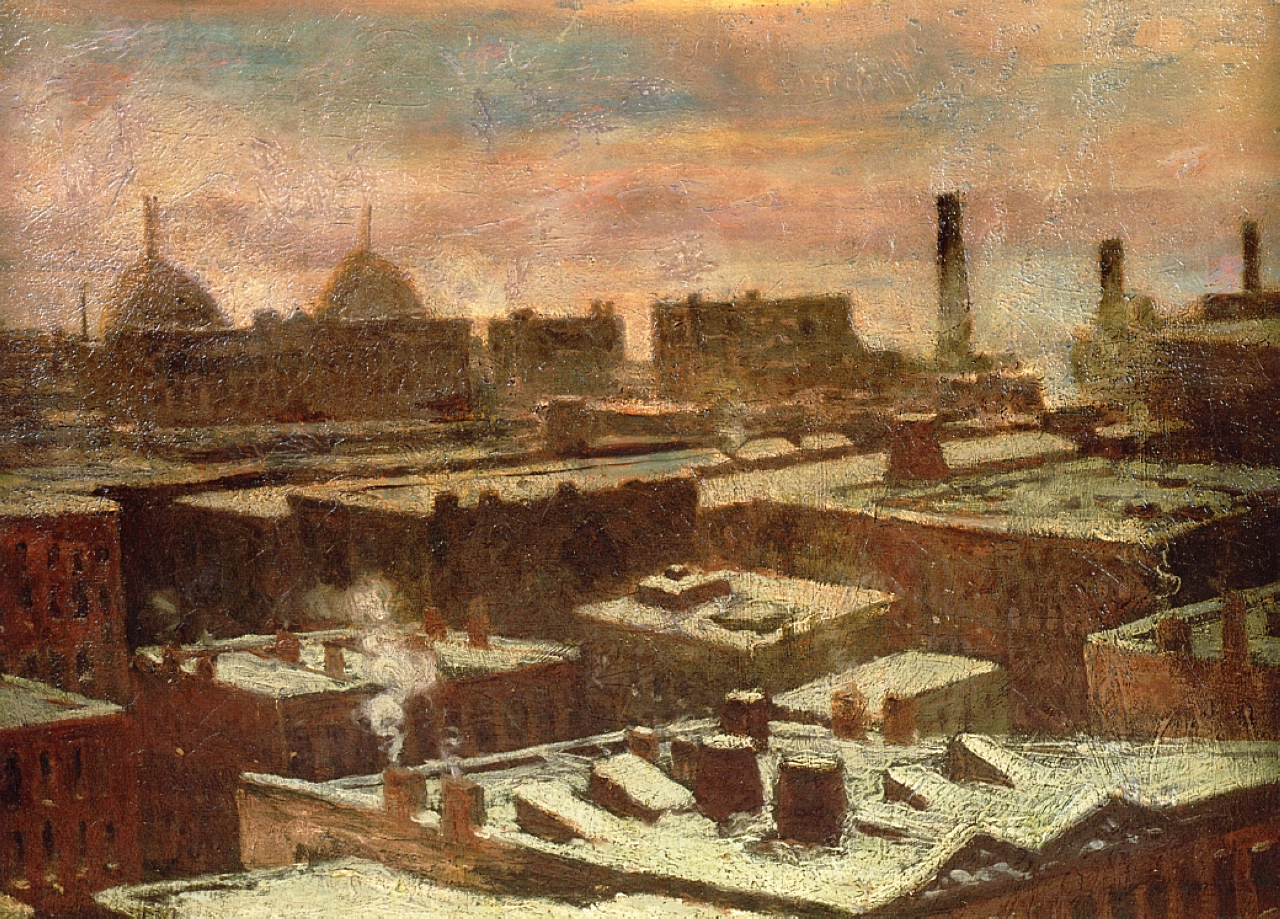In this hand-painted canvas image, the scene captures the rooftops of an old, industrial European city, possibly in England. The predominant color palette consists of browns and beige, evoking a sense of age and wear. The rooftops are dotted with smoking chimneys and old structures, showcasing signs of decay such as tiles lifting off and paint cracking. The buildings, made primarily of red brick, appear worn and dirty, accentuating their antiquity.

Towards the background, the skyline features several towering smokestacks, suggesting the presence of factories, while further back, two domes with spires add a touch of architectural elegance. The sky above is a muted blend of pink, orange, and blue, merging together in an overcast haze that accentuates the city's somber and faded atmosphere. The painting itself shows signs of aging, adding to the historic and nostalgic feel of the scene.